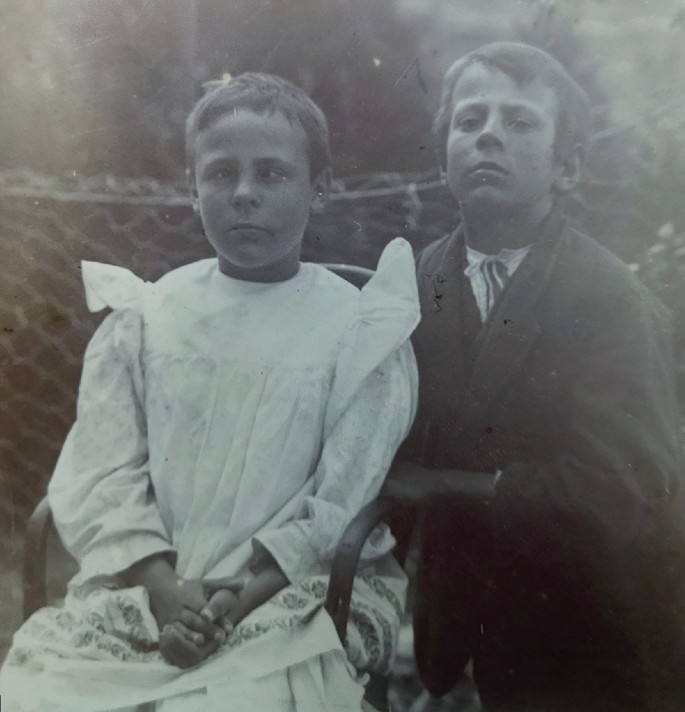In the center of this black-and-white vintage photograph, two children with fair skin and short hair are portrayed in striking detail, suggesting they could be siblings. The child on the left, seated in a chair, is adorned in a light-colored dress with floral patterns around the hem and puffed sleeves, exuding a quaint charm. Her slightly crossed eyes and folded hands rest solemnly in her lap, adding a poignant touch to her expressionless face. Next to her, a boy kneels to match the chair's height, his hand resting gently on the armrest. He is dressed in a dark jacket with a white shirt underneath, his hair parted neatly, and his chin lifted slightly. Both children hold a serious demeanor against a blurred, gray backdrop, capturing a moment frozen in time.